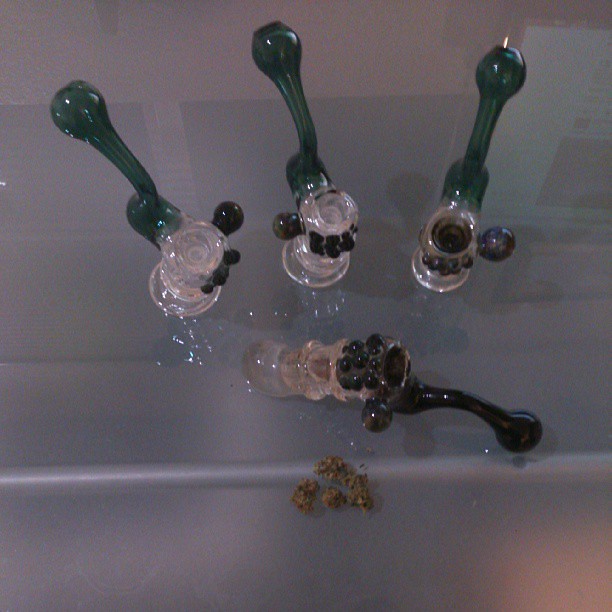The image features a collection of glass drug paraphernalia, likely used for smoking marijuana or other substances. The scene is set on a glass surface, displaying four primary pieces. Each piece has a bulbous top that narrows and widens toward the bottom. Three of these pieces stand upright, showcasing a striking aquamarine or dark teal blue color on their bulbous ends, with clear glass bodies that incorporate black and various other colors. The fourth piece, distinct with its curved handle and black bulb, lies horizontally at the bottom of the image. The glasswork of this particular piece appears more disheveled. Additionally, the surface around the items contains some brown residue and possibly droplets of glass or water, contributing to a cluttered, intricate scene that leaves a strong impression of disarray and usage.